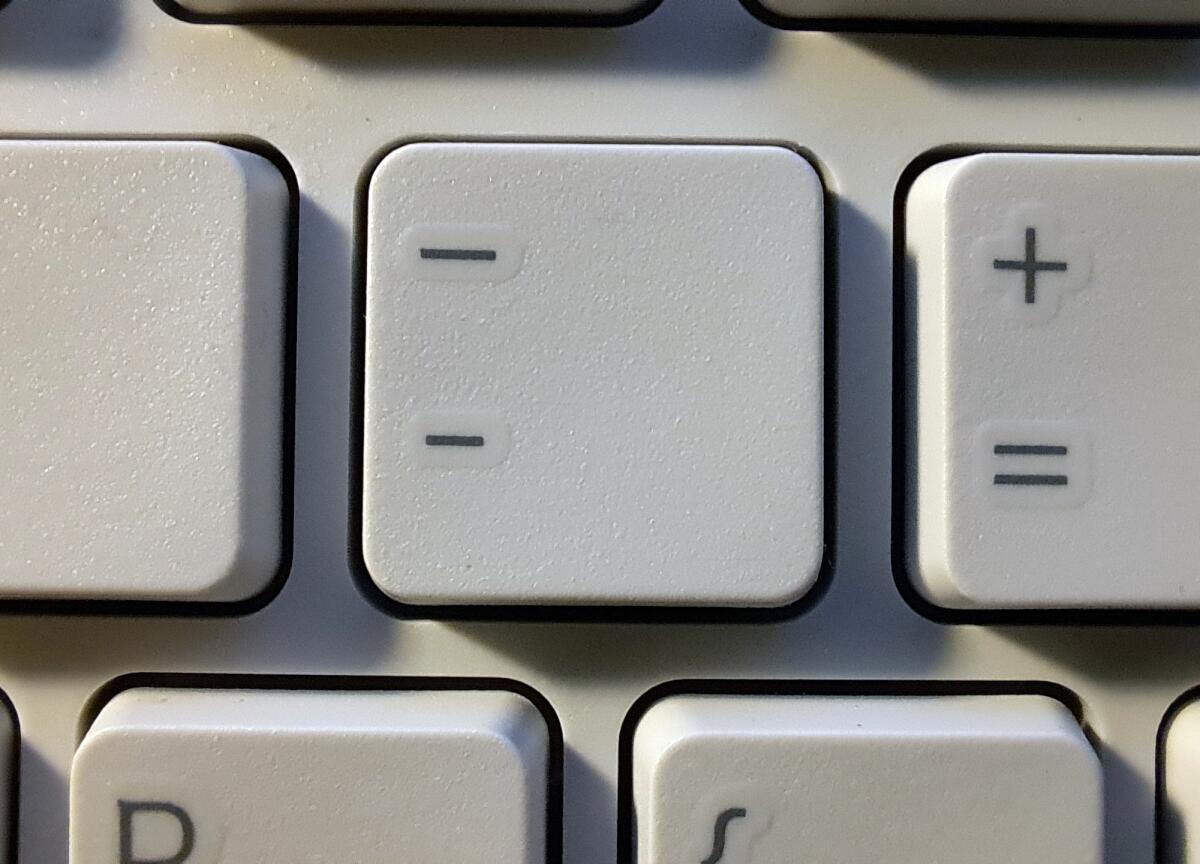This close-up image depicts an eggshell white computer keyboard focusing on the dash key, which transforms into an underscore when the shift button is pressed. This key is centrally placed in the photo and is the only fully visible key. To the right, the photo captures part of the key with a plus sign and an equal sign. The image also includes partial views of the surrounding keys: the tops of the P key and the open bracket key below, and segments of three keys in the row above. The keyboard features light gray keys marked by black symbols.